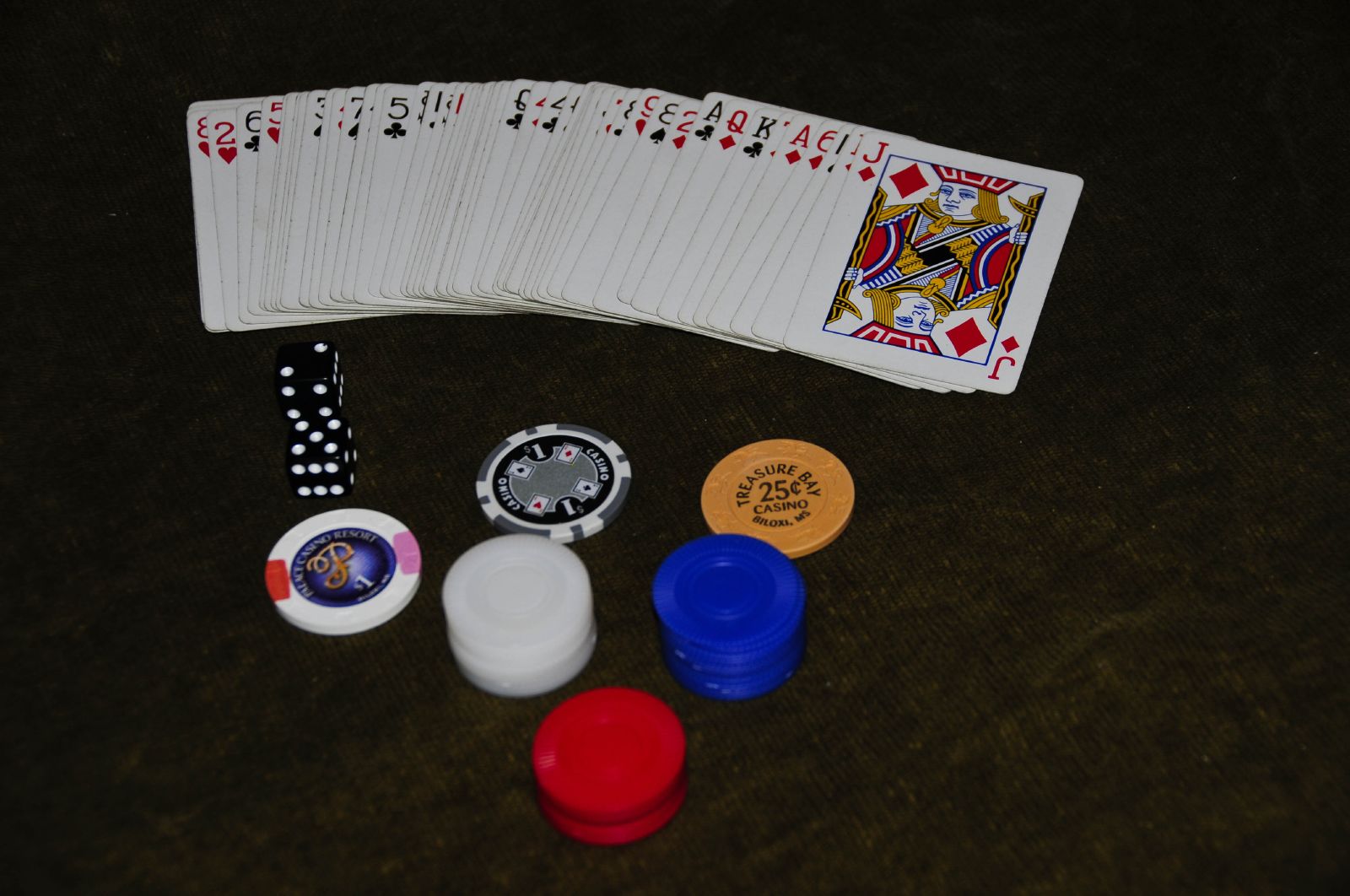A deck of playing cards is meticulously arranged in a domino effect on a sleek, black wooden surface. Each card is clearly visible, displaying a variety of suits: clubs, hearts, spades, and diamonds. The sequence concludes with a jack of diamonds prominently at the end of the line. Adjacent to the cascade of cards, two black and white dice are positioned, either beside or slightly below the playing cards. Accompanying these are several gambling chips in six distinct colors and designs, including white, blue, red, and three other unique varieties. The scene evokes a sense of anticipation and excitement, characteristic of a high-stakes game night.